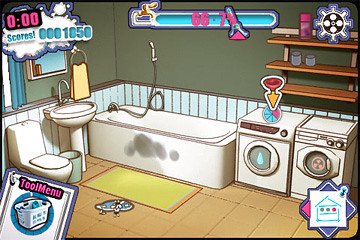A detailed screenshot from a simple mobile game or application, featuring a cartoon-style illustration of a bathroom. The left side of the image shows a neatly drawn toilet and sink. Center frame, a bathtub stands prominently, marred by noticeable black smudges, hinting at a cleaning objective for the player. On the right side, a washing machine and dryer are depicted, complete with shelves above stocked with various laundry supplies. The game environment is further detailed with the addition of a bath mat and a small puddle of water in front of the bathtub, adding to the interactive elements likely involving cleaning tasks.